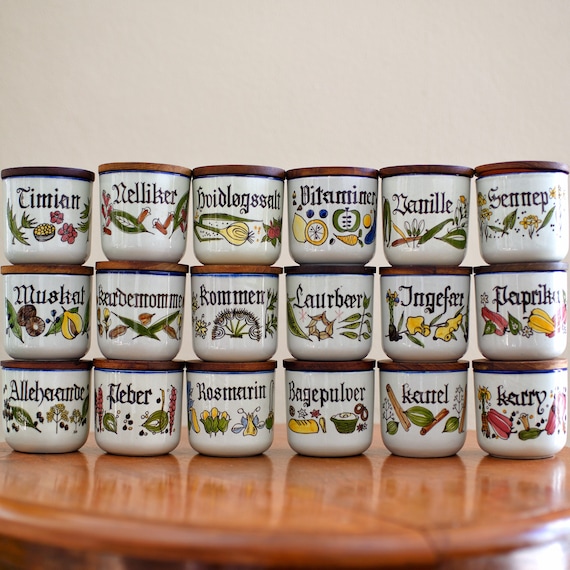This image displays 18 white porcelain jars, each adorned with a brown wooden lid, arranged neatly in three rows of six on a brown wooden table. Each jar features intricately designed illustrations of various foods, such as fruits, vegetables, breads, and corn, each depicted in vibrant colors—red peppers, yellow peppers, yellow corn, and brown bread. The jars are labeled with names that, while unfamiliar, suggest they could be spices or food items, written in an old-style script. Notable terms include "TIMIAN," "VITAMINER," and "BAGEPULVER," accompanied by images such as bread being dipped in a sauce and a homemade pretzel. The labels and designs hint at their possibly German or other foreign origin, adding a touch of cultural flair to the display.